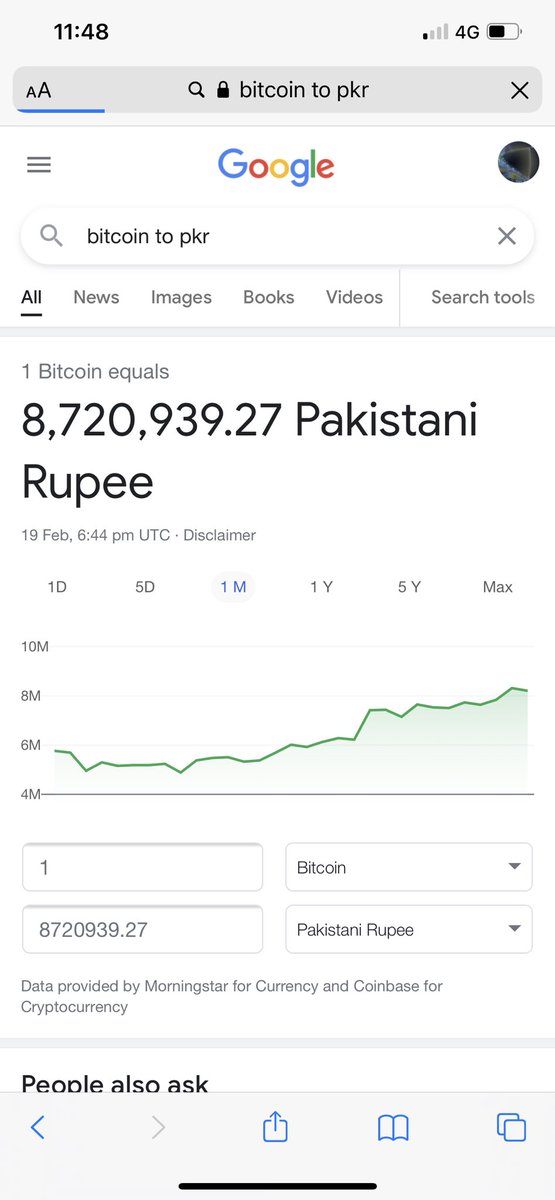The image showcases a Google search being viewed on a mobile device. In the upper left-hand corner, the time is displayed as 11:48. The upper right corner shows a signal strength of one out of four bars, a 4G icon, and a half battery life icon. Below the address bar, which contains an AA logo on the left and a search term “Bitcoin to PKR” with a close (X) button on the right, there are standard browser icons: three horizontal bars for more options on the left, a profile image on the right, and the Google logo in the center. 

Directly below the Google logo is a search bar with the term “Bitcoin to PKR” entered. Beneath this are navigation options including ‘All’, ‘News’, ‘Images’, ‘Books’, ‘Video’, and ‘Search tools’, with ‘All’ currently selected. The search results indicate that 1 Bitcoin equals 8,720,939,027 Pakistani Rupees, with the data timestamped at February 19, 6:44 PM UTC. A disclaimer mentions that the data is provided by Morningstar for currency and Coinbase for cryptocurrency. A one-month graph spanning from the 4th to the 10th of the month shows a steady increase in Bitcoin's value, represented visually beneath this information.